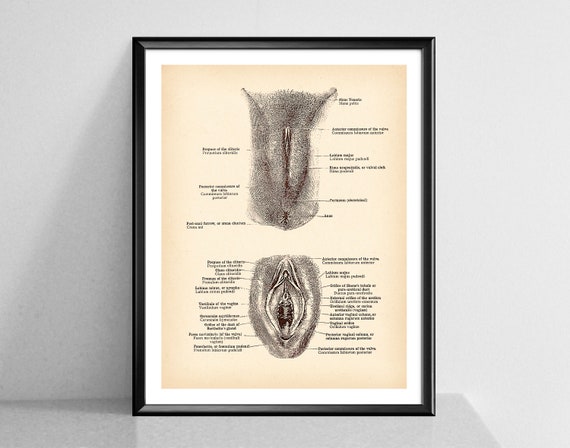This detailed digital print, evoking the style of a vintage medical anatomy textbook, is presented within a black picture frame. The solid light beige background of the print is bordered by a white photo mat, adding a crisp contrast before meeting the black frame. The framed print is propped upright against an off-white to gray wall, perched gracefully on a visually blending ledge or table. The artwork meticulously illustrates two detailed anatomical sketches of women's genitalia, displayed one above the other. Multiple fine lines extend from various parts of the sketches to corresponding labels, identifying each anatomical feature. Although the labels are too small to be read clearly, the print showcases an abundance of detailed annotations, likely numbering around twenty, focused on various aspects of the genital anatomy. The composition and meticulous detail suggest it is the type of medical illustration that could adorn the walls of a doctor's or gynecologist's office, offering a clean and educational visual aid.